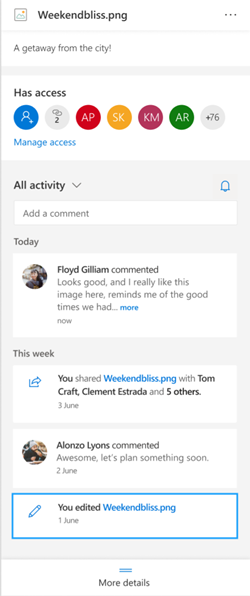The image is a vertical rectangle, likely captured from a mobile app interface. At the very top, the file name "weekendbliss.png" is displayed, followed by the phrase "a gateway from the city." The overall background of the image is predominantly white. 

Just below the header, there is a section labeled "Access," which features six colorful icons arranged horizontally from left to right, and an option labeled "Manage Access."

Proceeding downward, a gray box titled "All activity" is accompanied by a downward-pointing arrow and a notification symbol on the far right. Below this, a white box is labeled "Add a comment," accompanied by an entry stating: "Today, Floyd Gilliam commented: 'It looks good and I really like this image here reminds me of the good times we had.'"

The section titled "This week" follows next, displaying another white box indicating: "You shared weekendbliss.png with Tom Kraft, Clement Estrada, and five others."

Further down, a small circular image appears, identifying an individual: "Alonzo Lyons commented: 'Awesome, let's plan something soon.'"

The final box states: "You edited weekendbliss.png on June 1st." 

Concluding the image, a link at the bottom reads "More details."